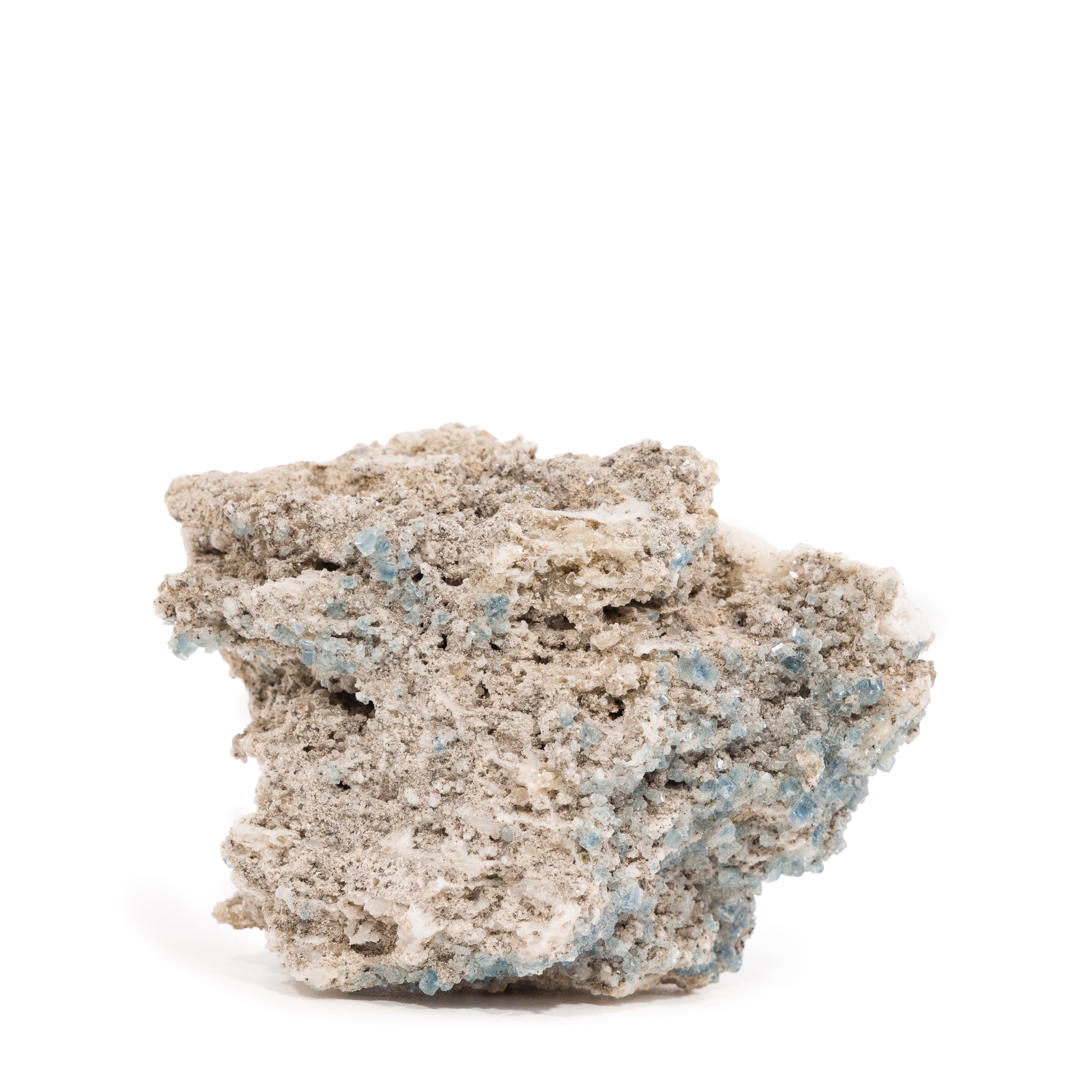This is a detailed close-up color photograph of a mineral specimen, often mistaken for other tiny objects. The rock features a combination of tan, gray, and light baby blue colors, with the blue areas consisting of tiny square crystals. The mineral is likely celestine (or celestite), which bears some resemblance to blue calcite. The rock is set against a stark white background and has a jagged, irregular shape. Despite its intriguing crystal formations, it's not considered a particularly attractive specimen and isn't highly valued.